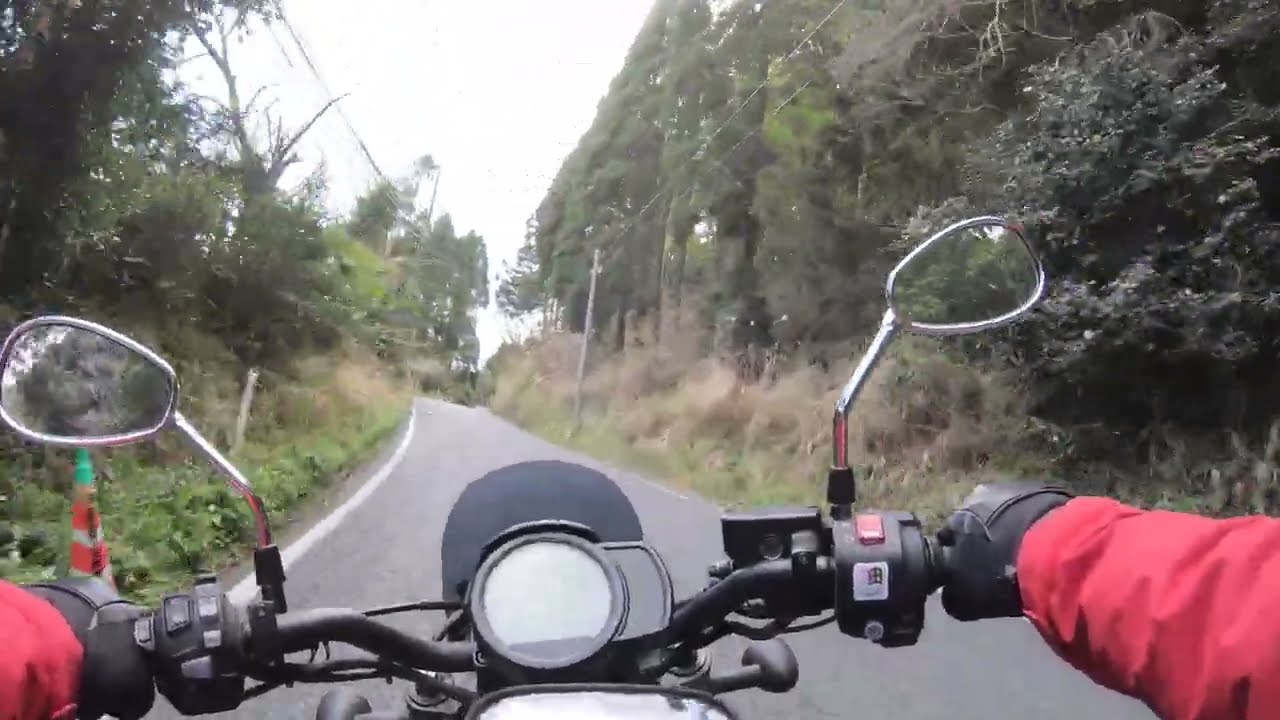This horizontally aligned rectangular image captures a slightly blurry, first-person perspective from a motorcycle rider traversing a narrow, gray-paved road with no visible center lines. The scene depicts the rider's forearms clad in a red jacket and black leather gloves, gripping the black handlebars of the motorcycle. Only the rider's hands, handlebars, and two silver side mirrors are visible, with all controls on the motorcycle being black except for a distinct red button on the right handle. The road is framed by tall grass and dense, dark green trees, with the right side appearing more heavily wooded than the left. Power lines run parallel to the road on both sides. A solid white line marks the left edge of the road, and there is a mention of an orange and white traffic cone positioned on the left side. The perspective directs the viewer straight ahead, down the narrow road flanked by lush greenery.